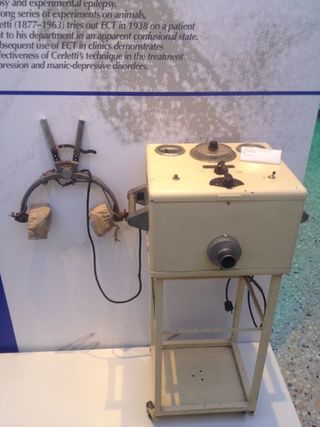This image showcases a very old antique electrical device alongside an equally aged set of headphones. The device, predominantly white and fashioned from tin metal, is mounted on a stand resembling a bedside table. The stand features a pale yellowish wood surface adorned with several burnt silver dials, including one prominent knob near what appears to be a drawer area. Situated on the wall behind the device, which also has wheels, is a museum placard with text that is difficult to read due to the muted purple background and black lettering. Select words are discernible, such as dates ranging from 1877 to 1961 and a reference to 1938, indicating the historical context and possible use of the device in electroconvulsive therapy (ECT) within clinics.

Alongside the machine, there is a blue dividing line on the placard that separates the top portion of the text from the lower section. Below this line, a pair of antique headphones is suspended on an upside-down V-shaped hook. These headphones, resembling old ice block tongs in design, have tan, marshmallow-like pads that are ancient and slightly ragged, evoking the visual of old, makeshift earpieces. A wire extends from the headphones, attaching to the side of the device, further solidifying its appearance as an old audio or telephone apparatus. An electrical cord is visible, hanging down from the rear of the device, though it is not plugged in. The device and headphones together paint a vivid picture of early electrical and audio technology, possibly linked to historical medical practices.